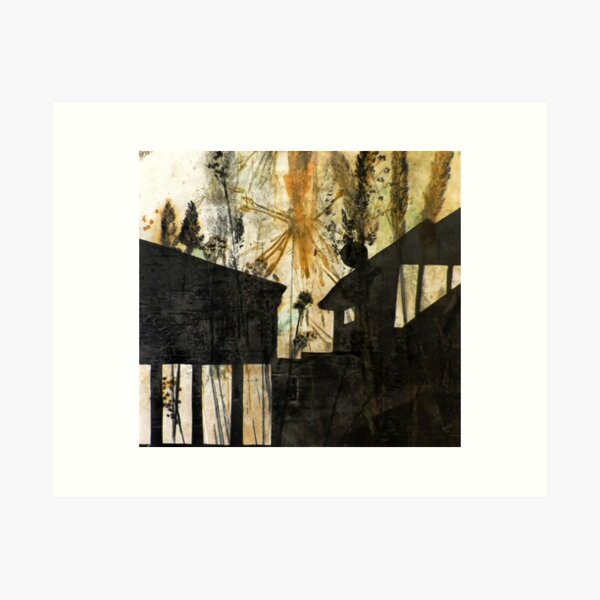This artistic image features a complex assembly of dark and neutral tones with a thick white border framing the scene. The painting itself presents an enigmatic mixture of objects and shapes set against a cream-colored background. Prominently, there are two heavily shaded structures: the one on the left is large and rectangular, somewhat resembling a billboard with three vertical legs descending from it, while the one on the right is reminiscent of a house, complete with silhouettes that could be interpreted as windows. Interspersed throughout the background are forms that vaguely resemble trees or stocks of grain, featuring long vertical sticks with feather-like leaves emerging from them, adding to the abstract organic feel. Central to the composition is an orange, dimly explosive, flower-like shape that introduces a burst of color, seemingly radiating from the center. The overall effect is a shadowy, atmospheric image, rich with ambiguity and open to interpretation.